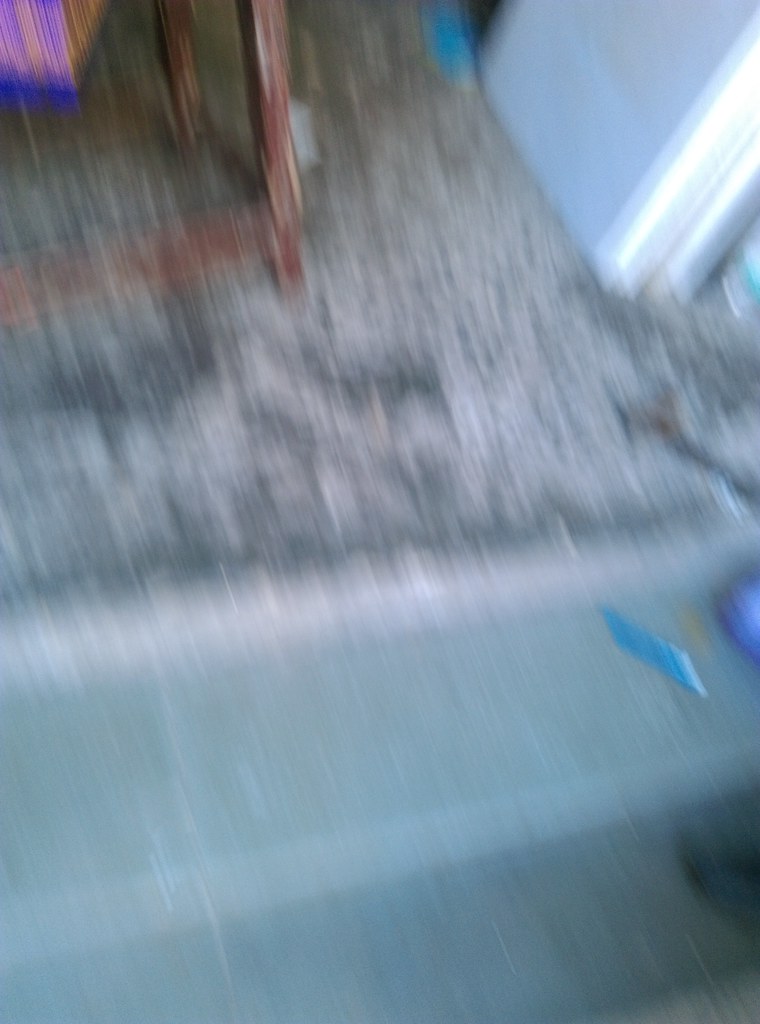This out-of-focus, low-quality color photograph seems to capture an indiscernible scene, possibly taken inside a residence, though there are mixed indications suggesting it might be outside. The blurred image is at a tilted angle, further complicating the interpretation. 

In the lower part of the frame, there are two wooden stool legs, dark brown and notably scratched, along with a brace that connects them. The ground below appears cement-like, characterized by a mix of slate grey and light grey, possibly a sidewalk. There's also a blue object in the lower right and rounder blue object in the upper right section. The background is marked by a white wall or molding in the upper left corner and a greyish side of a building in the upper right.

Interspersed with these elements are patches of dirt and perhaps a bit of grass, suggesting an outdoor vibe. Additionally, a blurry pink square with a strip of royal blue appears in the upper left, and another square object in blue and yellow can be seen. Throughout the shot, reflected light spots are noticeable, adding to the chaotic and out-of-focus nature of the photograph.